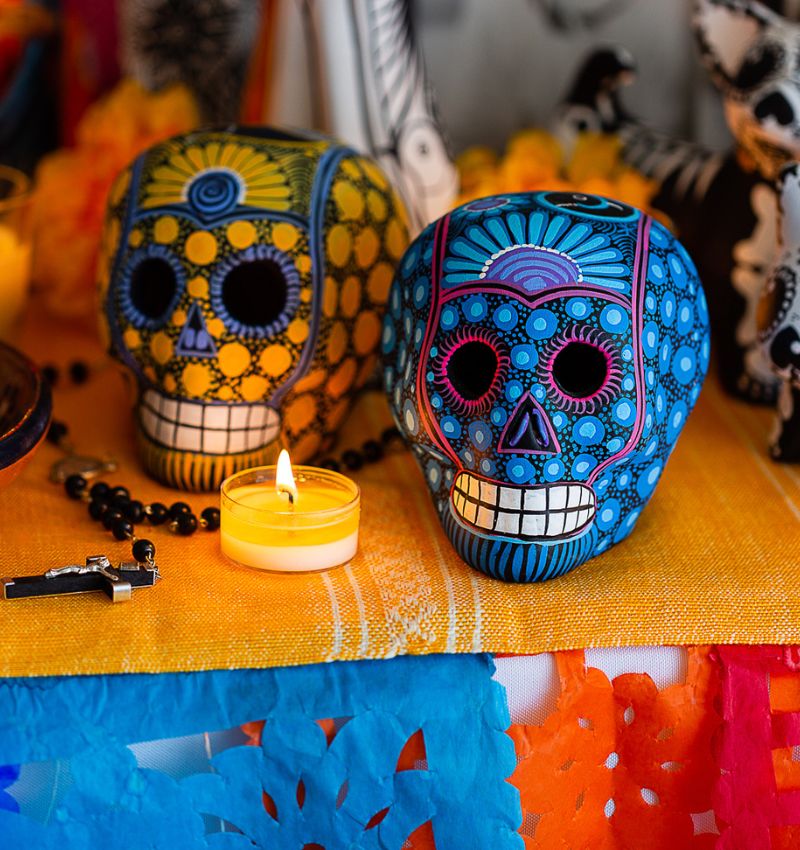The image showcases an elaborate and colorful display likely intended for a festive occasion such as Halloween or a cultural celebration. Central to the scene are two stylized, decorative skulls placed on a table that is carefully adorned. The table is draped with an orange cloth and overlaid with intricate cut-out papers in shades of blue, orange, and pink. 

On the left, a yellow skull with black accents and blue stripes around its eyes faces the camera. Its dark black eyes and prominent white teeth create a striking contrast. Adjacent to it is a blue skull peppered with light blue circles and trimmed with pink details extending from the crown down to the mouth, also featuring dark black eyes bordered with pink and vivid white teeth.

A yellow-and-white lit candle is positioned between the skulls, enhancing the setting's ambiance with its flickering flame. To the left of the candle lies a rosary, draped around the yellow skull. The intricate paper cut-outs below the tablecloth add a delicate texture to the overall composition. In the blurred background, additional decorative elements and possibly flowers contribute to the festive atmosphere.